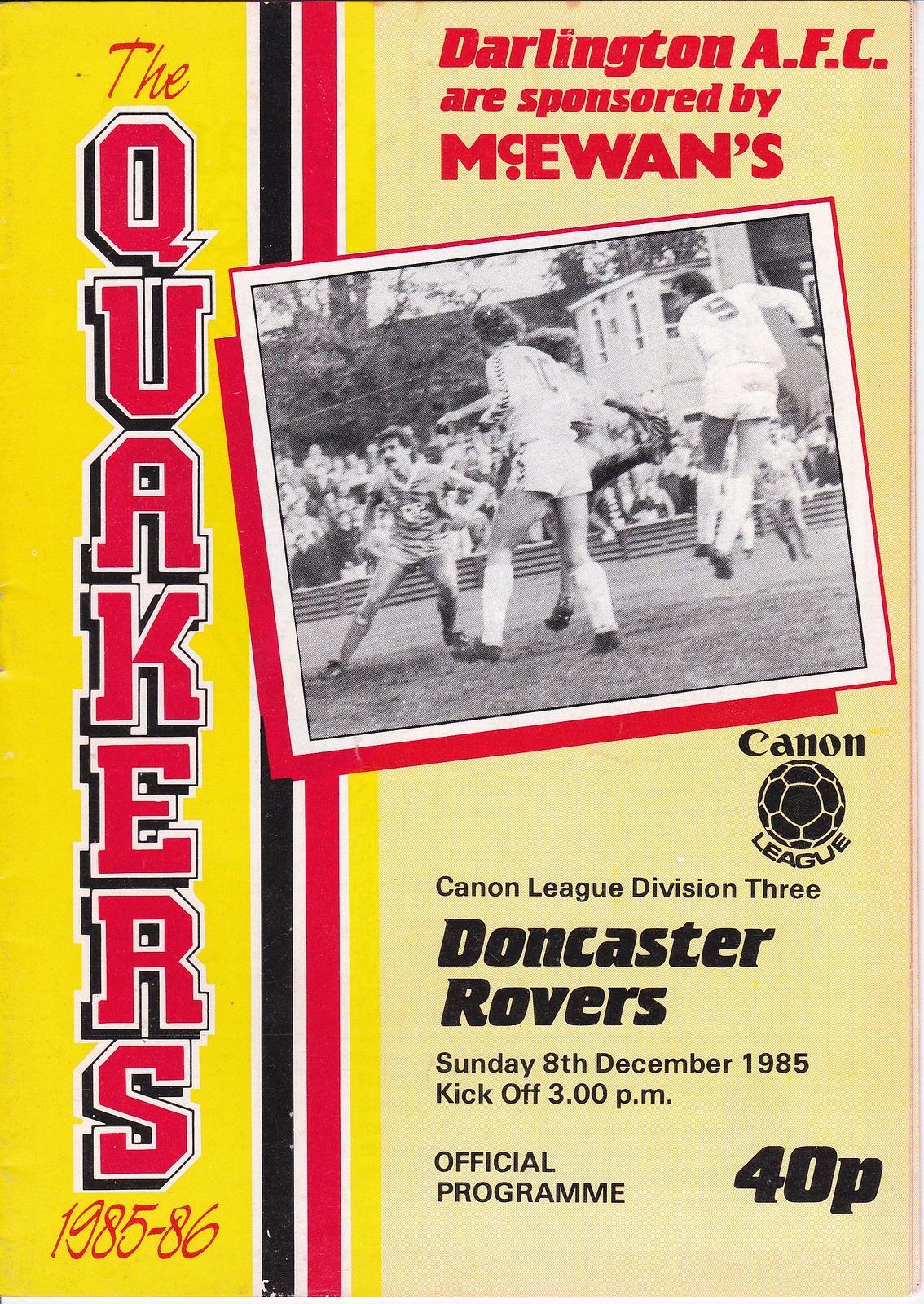The cover of this official program for an English League soccer match, featuring Division III team Darlington AFC, is predominantly yellow with bold red and black accents. At the top right, in red text, it reads “Darlington AFC,” sponsored by McEwan’s. Vertically down the left side, in large red letters against a yellow background, it states "The Quakers, 1985-86." The central portion of the cover displays a black-and-white photograph of soccer players engaged in a match at a smaller outdoor stadium, with a visible number 9 player jumping in the air. Underneath the photograph, in black text, it reads “Cannon League Division III,” alongside a logo of a soccer ball. Below this, in black letters, it details the upcoming game: “Doncaster Rovers, Sunday, 8th December 1985, kickoff, 3 p.m.” Toward the bottom right, it mentions "Official Program" and "40p" in bold black letters.